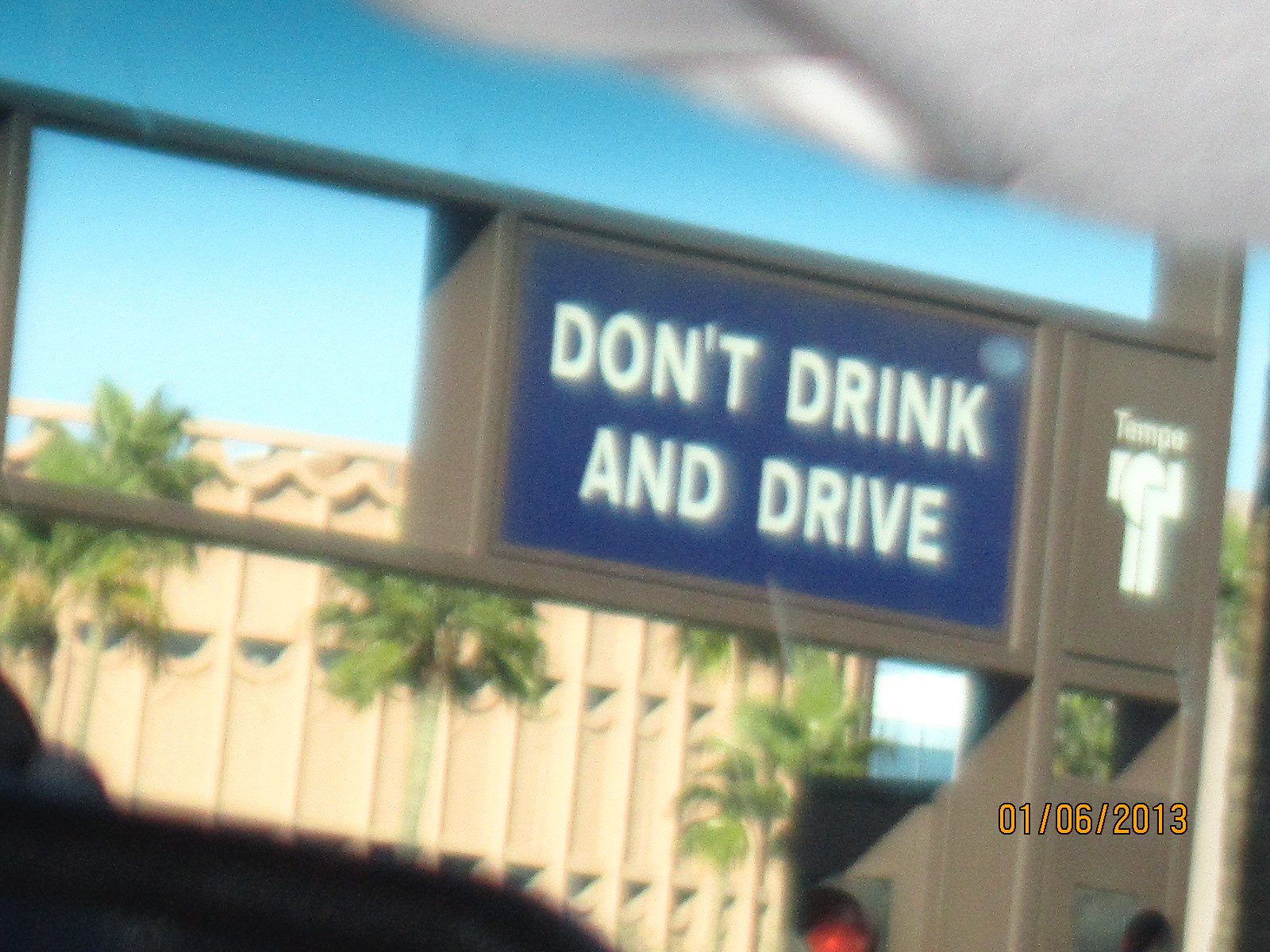The photograph, presumably taken from a moving vehicle or dash cam, depicts a slightly blurry scene set outdoors on a clear day, marked by a turquoise blue sky transitioning into white near the horizon. In the bottom right corner, there is a small orange date stamp reading "01-06-2013." Central to the image is a roadside sign featuring a blue banner with the prominent white text "Don't Drink and Drive." Adjacent to this banner on the sign, there is an unclear city name that could be either "Tempe" or "Tampa," along with a bold white T-shaped logo below it. The sign is mounted on a robust pole with a grey-brown frame. In the background, a tan fence can be seen, partially obscured by slim tropical trees with pointy green leaves, adding a touch of greenery to the setting.